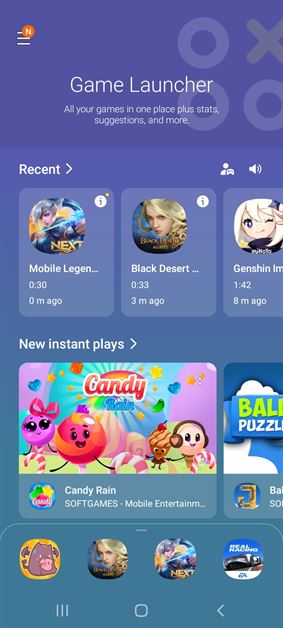A vertical screenshot from a smartphone showcasing the Game Launcher interface. The background transitions from a purple gradient at the top to an aqua greenish-blue at the bottom. Dominating the top of the image is a dark purple section with white text that reads, "Game Launcher. All your games in one place plus stats, suggestions, and more." This section features an X and O pattern as a backdrop, giving it a playful aesthetic. In the upper left-hand corner, there is a small menu icon comprising three horizontal lines and an adjacent circle with the letter "N".

Beneath this, the interface displays three recently played games: Mobile Legends, Black Desert, and Genshin, each represented by vibrant character images within boxes. Further down, white text announces "New Instant Plays," under which two games are highlighted. On the left is "Candy Rain" by Soft Games, featuring a pastel-colored animated illustration. To the right, slightly cut off, is "Ball Puzzle." 

At the bottom of the screen, four game icons are shown, each representing different games, flanking three navigation buttons, standard on many smartphone interfaces. The overall design is user-friendly and visually appealing, with a seamless gradient enhancing the aesthetic appeal.